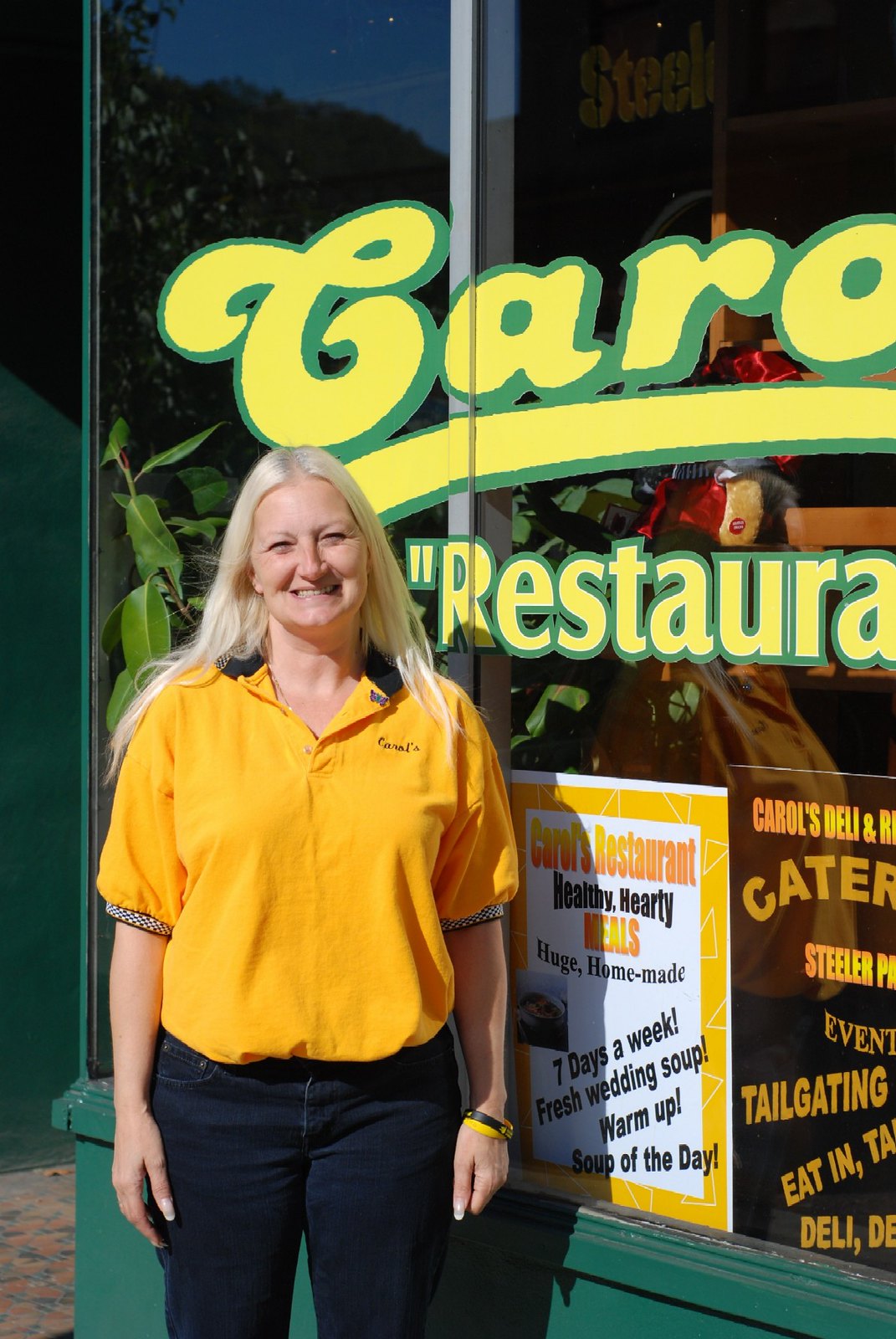In the photograph, a woman with long white-blonde hair stands smiling toothily in front of the window of Carol's Restaurant. She is wearing a short-sleeve button-up shirt, likely with 'Carol's' written on it, paired with dark denim jeans and a yellow Livestrong bracelet on her wrist. The window behind her prominently displays painted yellow text with a green border reading "Carol's Restaurant." Below this, a white poster with an orange border reads "Carol's Restaurant" in orange, followed by "Healthy, Hearty Meals" in black, "Huge Homemade" in orange, and a photograph of a bowl of soup. The poster also lists "Seven Days a Week, Fresh Wedding Soup, Warm Up, Soup of the Day" in black text. To the right, partially visible, is a black poster with some text cut off, mentioning "Carol's Deli" and services related to catering and tailgating. The scene is captured in bright daylight.